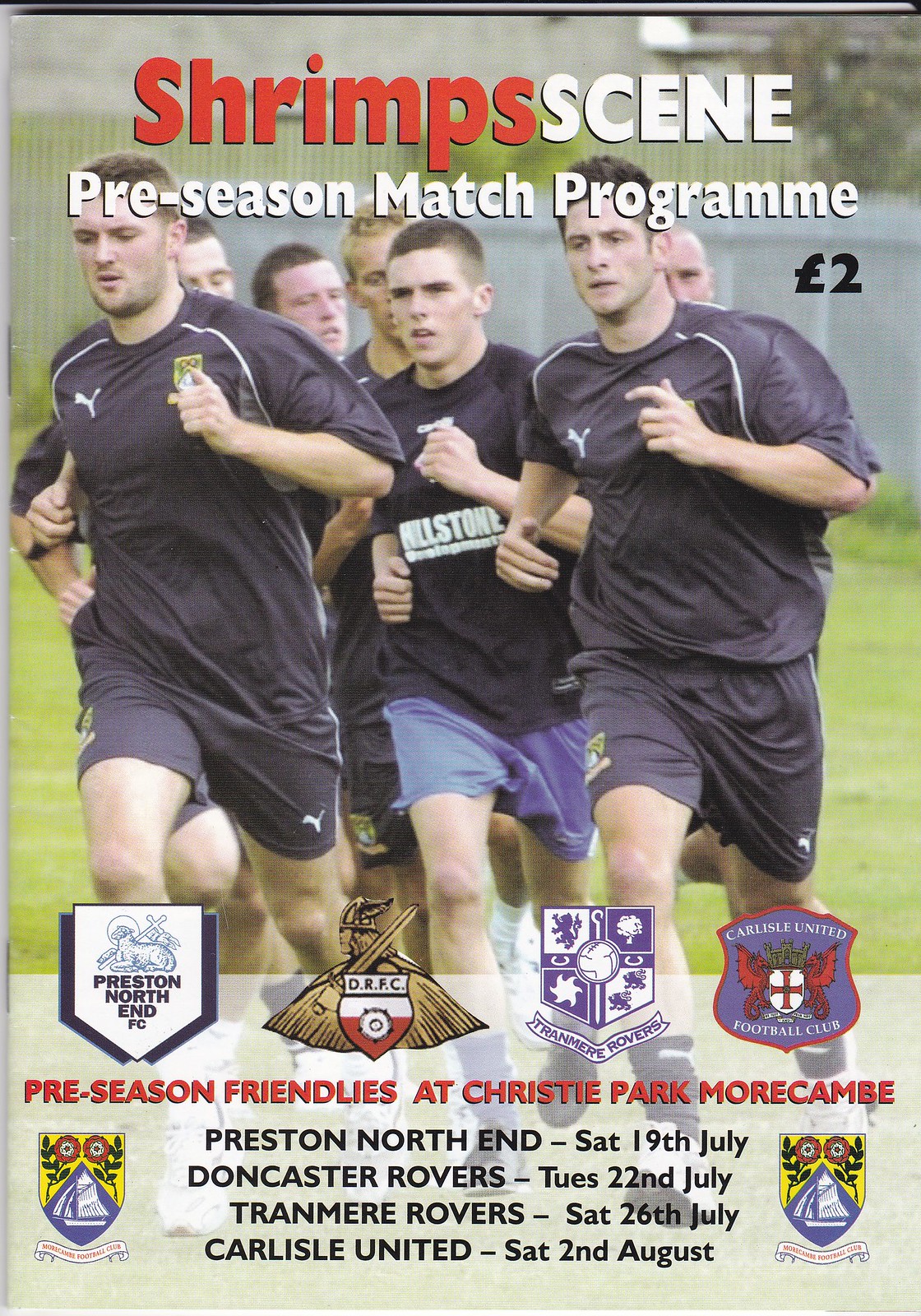The image is a cover of a football preseason match program titled "Shrimps Scene Preseason Match Program," priced at 2 Euros. The scene features young men in navy blue shirts and shorts running on a green field. The program lists "Preseason Friendlies at Christie Park, Morecambe," with detailed match dates, including Preston North End on Saturday, 19th July; Doncaster Rovers on Tuesday, 22nd July; Tranmere Rovers on Saturday, 26th July; and Carlisle United on Saturday, 2nd August. Below the running athletes, there are various football club crests, including those of Preston North End, Doncaster Rovers, Tranmere Rovers, and Carlisle United.